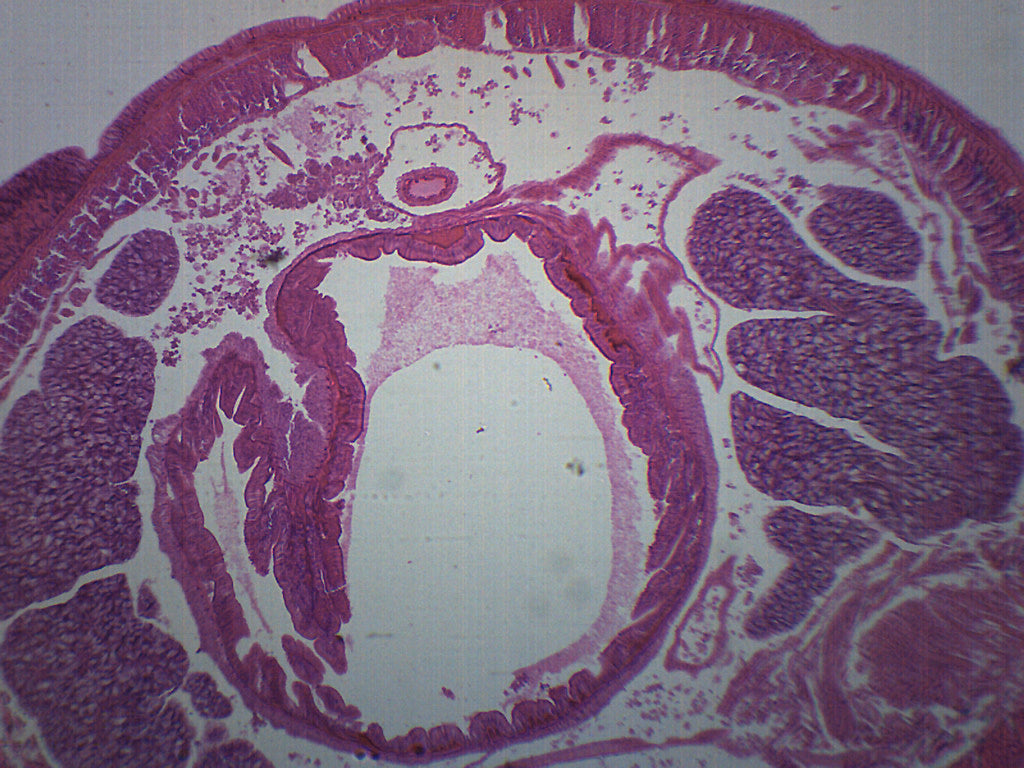The image presents an intriguing piece of abstract art that provocatively melds colors and textures on a white canvas background. Central to the composition is a deep maroon-pink circular form, which stands out amidst the scattered particles of dirt, debris, and other unidentifiable objects strewn across the canvas. This primary circle features a dark, uneven border with multiple maroon and purple splotches peppering its surface, suggesting an organic depth. Intriguingly, this form bears a divot on the left-hand side, disrupting its symmetry, and transitions into a lighter pink as it approaches the inner broad white circle at its core. The entire composition exudes a sense of modernity and spontaneity akin to spin art, where the paint appears to have been applied in an uncontrolled manner, creating a fluid, almost accidental pattern. This image could evoke the microscopic view of tissue or a cell, with its intricate details reminiscent of biological structures. Despite its abstract nature, the image is meticulously detailed, offering a feast of textures and colors that captivate the viewer's imagination.